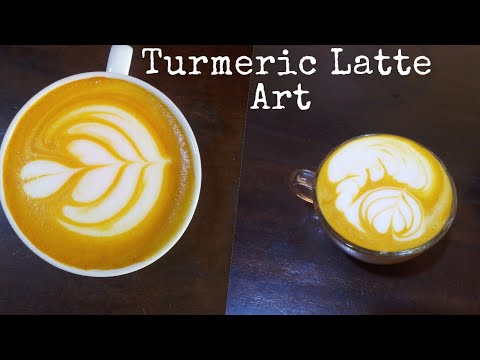In this advertisement for Turmeric Latte Art, a stunning image showcases two intricately designed lattes placed against a rich, dark-stained wood dinner table. At the top of the photo, the text "Turmeric Latte Art" is prominently displayed. On the left, a top-view of a white coffee mug reveals a perfectly crafted light brown latte topped with a delicate white cream design resembling a tulip with three sets of leaves. To the right, a clear mug holds a similarly colored latte with another floral pattern in white cream, though with a less defined bud and leaves. Both drinks exhibit a captivating mix of creamy white designs against a pumpkin-orange and coffee-hued backdrop, embodying the essence of turmeric latte artistry.